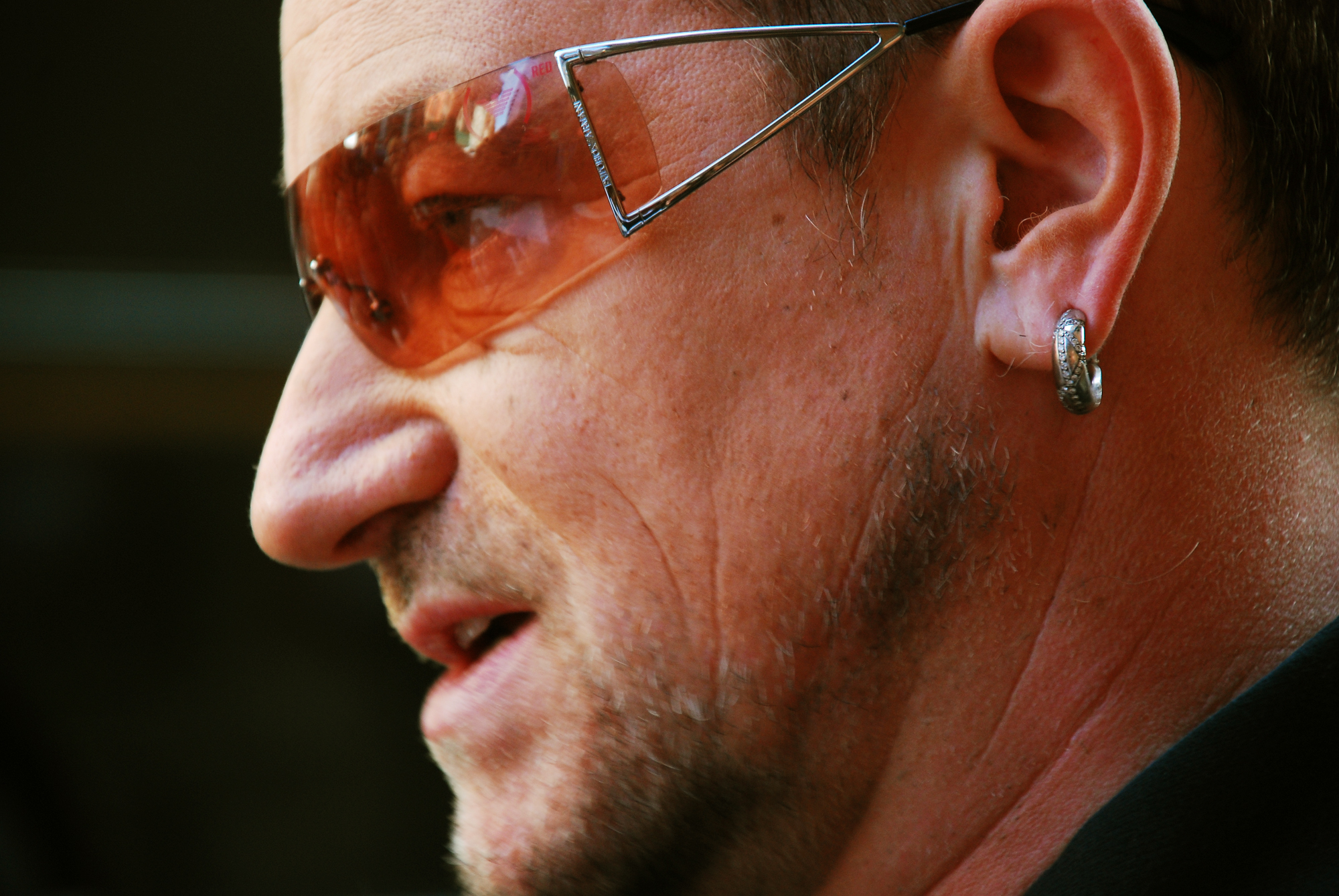The image is a detailed, up-close profile picture of the singer Bono. He is positioned on the right side of the screen, facing left, with a black background that makes it difficult to discern where the picture was taken. Bono sports distinctive orange-tinted sunglasses with metal frames that have a unique triangular design. He also wears a silver hoop earring with a design on his right ear. He has a short mustache and beard, along with visible smile lines and neck wrinkles, which are highlighted by the close-up nature of the photo. His hair appears dark, with noticeable sideburns. Bono’s mouth is slightly open as if he is speaking, and he wears a dark shirt or jacket that blends into the background.